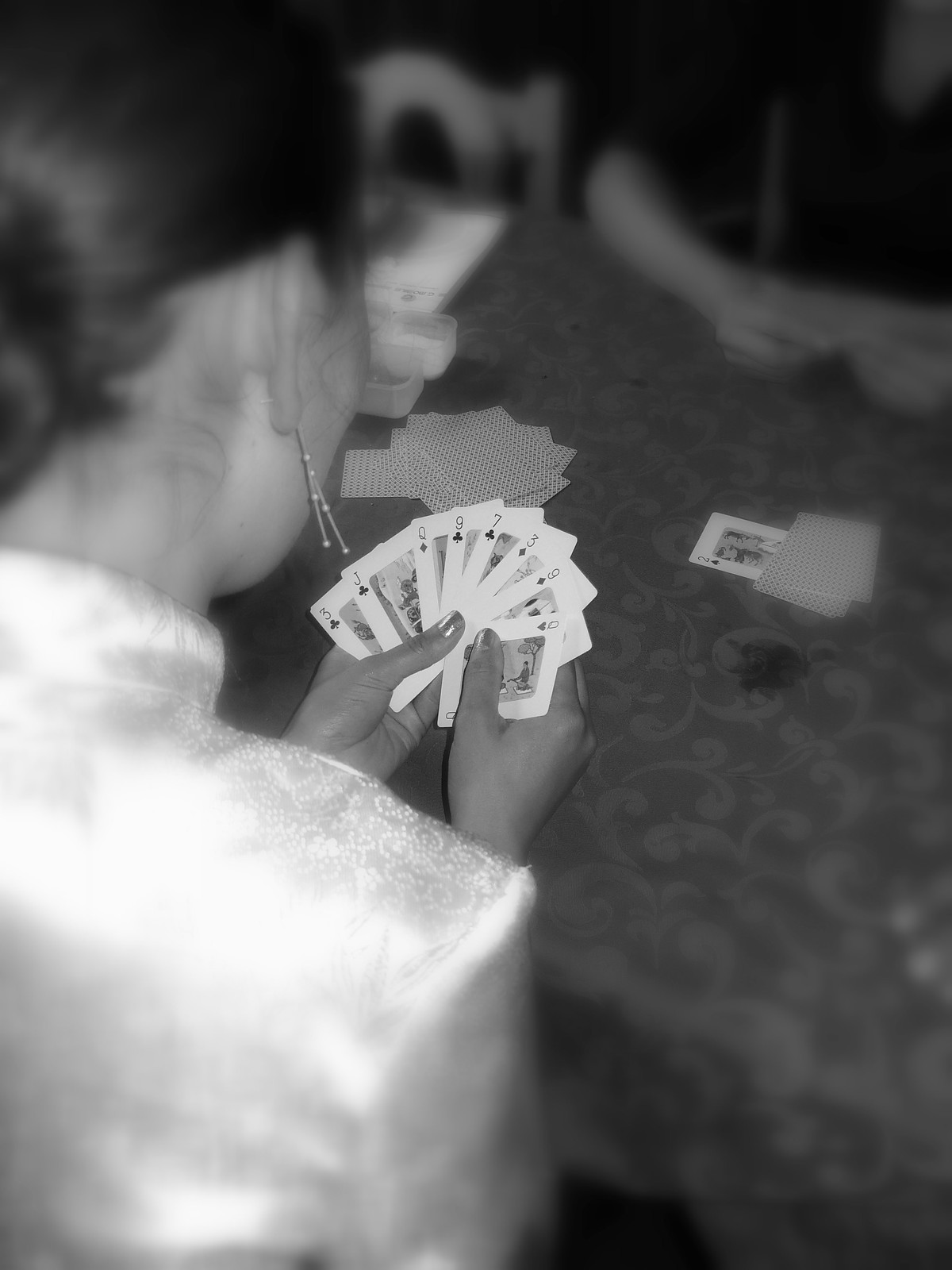In this evocative black and white photograph, we see a scene centered around at least two individuals engrossed in a card game. On the left-hand side of the image, a woman with her hair pulled back, wearing long earrings and a white top, is prominently featured. She holds a hand of cards that includes the three of clubs, the jack of clubs, the queen of spades, the nine of clubs, the seven of clubs, the three of spades, the three of diamonds, the nine of diamonds, and the queen of hearts. 

To the upper right of the image, there is a blurred figure, partially visible, whose indistinct hands suggest they are also holding cards. The table, adorned with a paisley-patterned tablecloth, has an array of cards scattered across its surface. Adjacent to the blurred figure, an empty chair is positioned, hinting at the possibility of additional players. Near the scattered cards, a small black stain is noticeable on the tablecloth. Among the cards on the table, two are facedown, while one face-up card revealing what appears to be the two of a certain suit. The photograph captures not just a game, but a moment brimming with engaging details and textures.